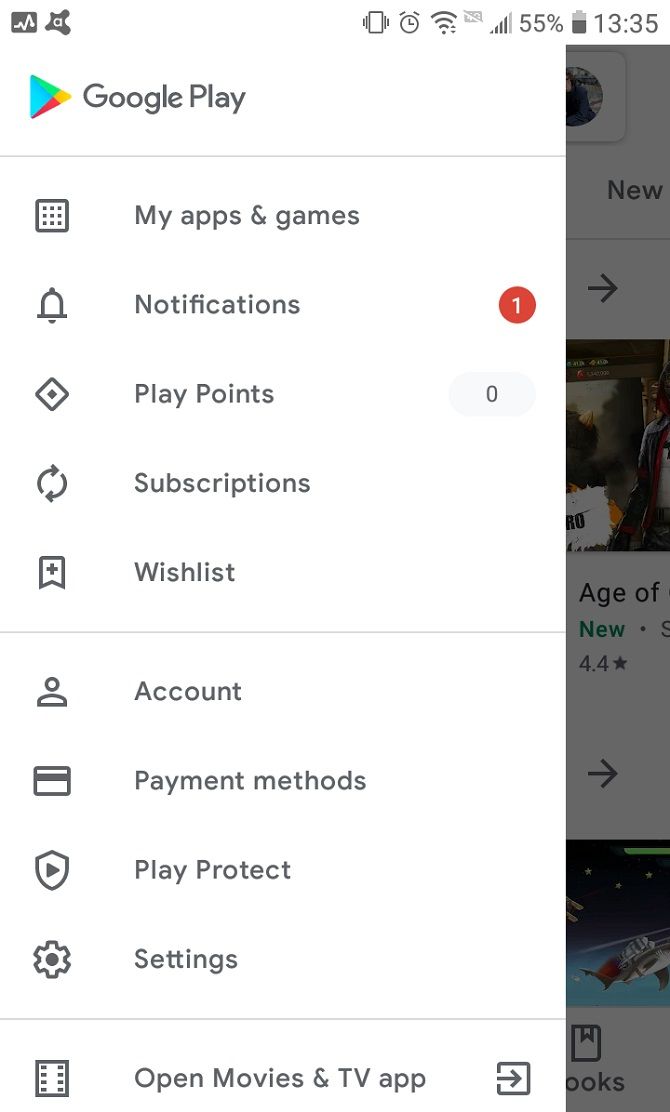The image is a screenshot taken from a tablet displaying the Google Play Store interface. At the top of the screen, the status bar shows various symbols and indicators: a timestamp of 13:35, battery at 55%, an 80% telephone signal, full Wi-Fi strength at 100%, and an active alarm icon. Below the status bar, the Google Play logo is visible, featuring a triangle with blue, red, green, and yellow colors, accompanied by a horizontal blue line underneath. Visible menu options include "My Apps & Games," "Notifications" (indicated by a red circle with the number 1), "Play Points," "Subscriptions," "Wishlist," "Account," "Payment Methods," "Play Protect," and "Settings." Each option is paired with a small representative icon on its left. At the bottom of the screen, there's an option labeled "Open Movies & TV App," signified by an arrow pointing to the right. The layout and icons are typical of the Google Play Store's organizational structure.